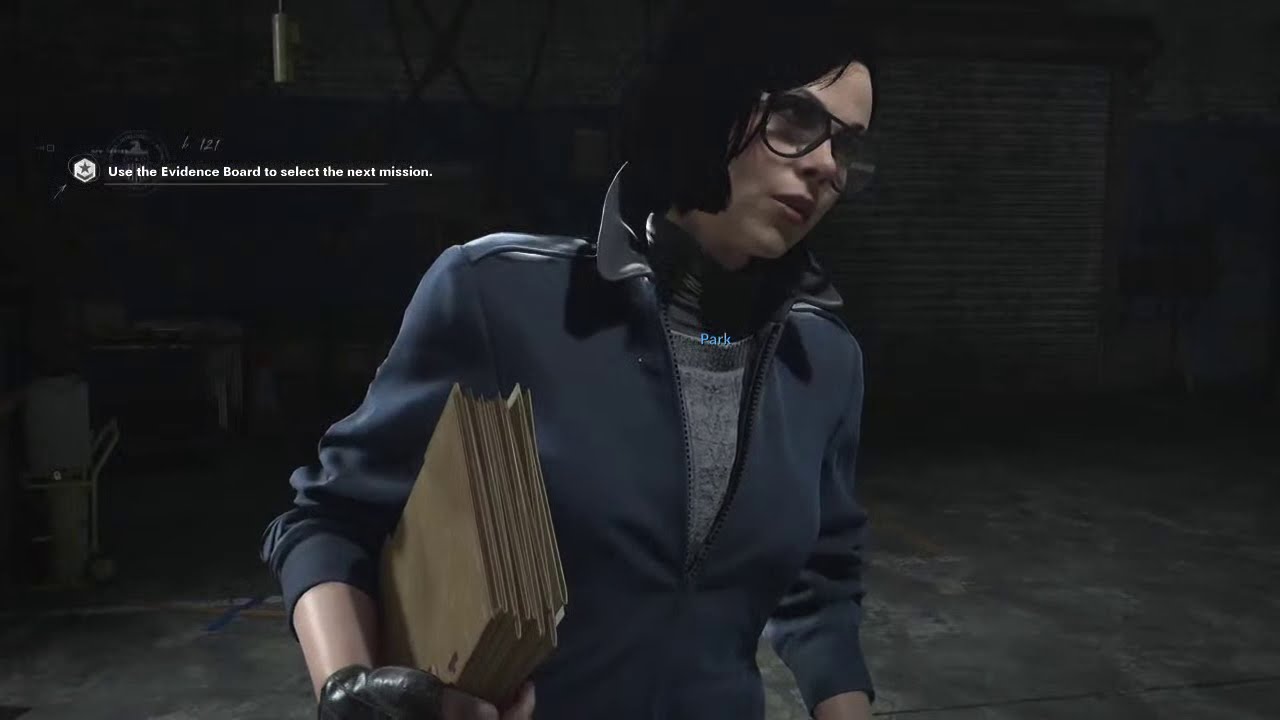In this detailed video game screenshot, a young woman stands prominently at the center of the frame, facing the roughly 5 o'clock position. She has shoulder-length black hair and wears black glasses, with a solemn expression on her face. Her outfit consists of an unzipped medium blue hoodie with rolled-up sleeves to her mid-forearms, revealing black gloves, and a gray shirt underneath. She holds a large vanilla envelope in her hand, suggesting a sense of purpose or distraction. The terrain beneath her appears to be gray pavement, possibly cement, and the background hints at an indoor warehouse setting with a grayish, chain-operated garage door partially visible on her left. In the upper left corner of the image, there's a directive text, accompanied by a star emblem, that reads: "Use the evidence board to select the next mission." The overall color palette of the scene includes shades of black, white, gray, tan, and various blues.